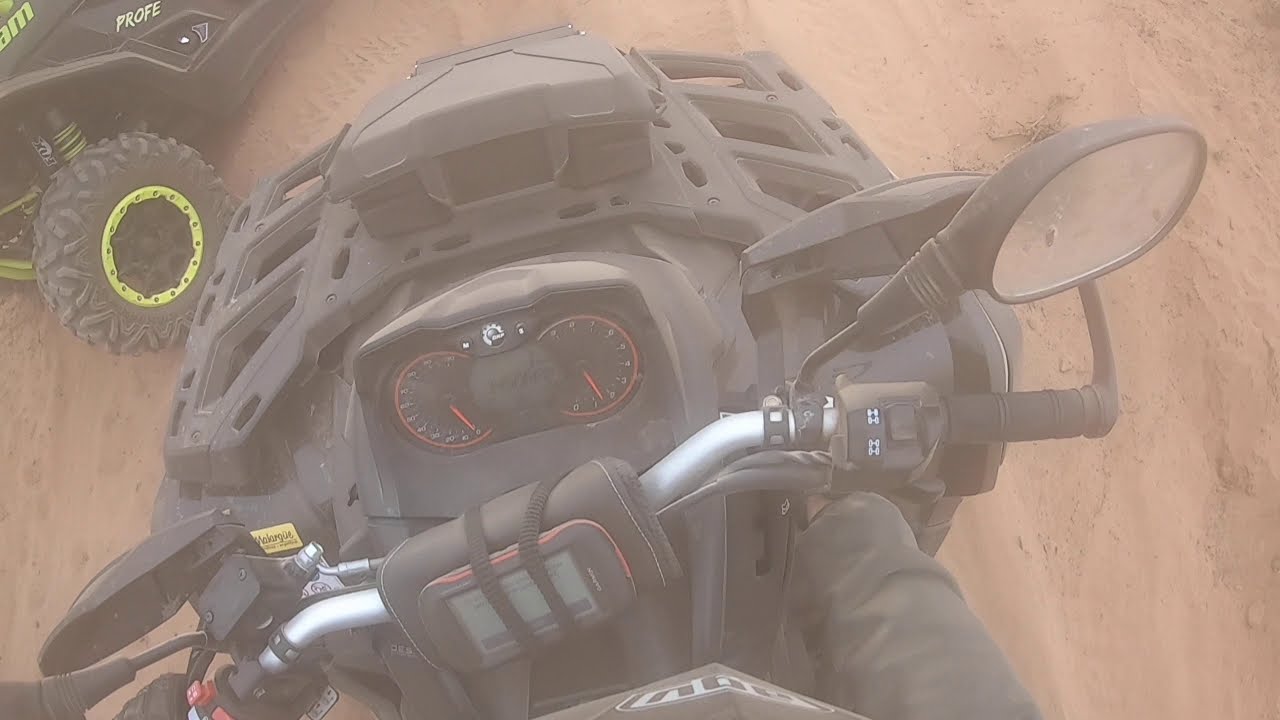Seen from a rider's vantage point, the image captures the handlebars of a black four-wheel ATV, or all-terrain vehicle, from what appears to be a head-mounted GoPro camera. The view looks down at the speedometer, tachometer, and a digital device mounted in the center of the handlebars. The rider's gloved hands gripping the handlebars are visible, and they seem to be wearing a leather coat. The scene is set on a tan, dusty dirt road. To the top left, another ATV partially enters the frame. This second ATV has black wheels with neon yellow rims, black spokes, and black springs with neon yellow coils. The word “PROFE” is painted on its side. The combination of elements—dusty terrain, the detailed and contrasting ATVs, and the dynamic rider's perspective—creates an engaging, action-packed snapshot of off-road adventure.